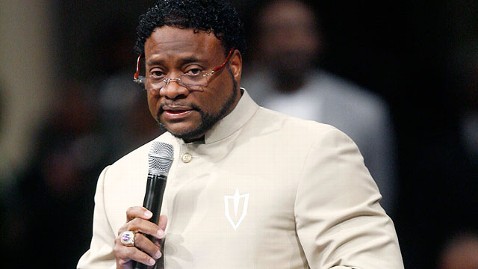A man with short black hair and glasses featuring red accents on the sides is looking directly into the camera. He sports a small black beard and is dressed in a tan jacket that extends slightly up his neck, secured at the collar with a button. A shield-like emblem adorns the left side of his jacket. In his right hand, he holds a black microphone with a silver top, while a large golden ring with a purple circular stone decorates his ring finger. The background is dark, with the blurred figure of another person visible.